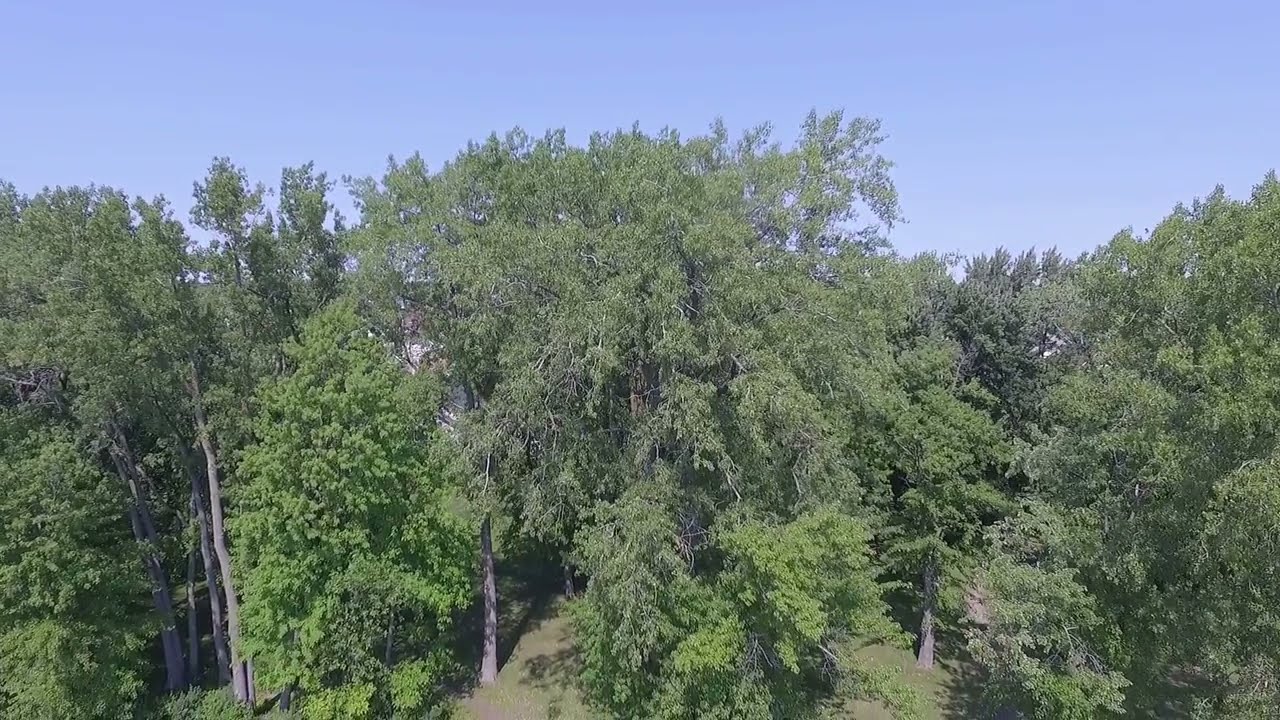The image captures a vibrant aerial view of a forest on a clear, sunny day. The sky above is a serene blue, entirely devoid of clouds, accentuating the lush green canopy below. The forest comprises a mix of tree species with thin, gray trunks that stand tall and relatively sparse, suggesting young or possibly recovering vegetation. The leaves range from lime green to forest green, giving the scene a rich tapestry of hues. Scattered shadows cast by the trees can be seen intermittently on patches of green grass and a narrow brown trail winding through the dense foliage. The overall impression is one of abundant greenery, with the foliage appearing almost bush-like, dense and varied in shade. The absence of clouds and the detailed shadows on the ground imply that the photo was likely taken at midday, capturing the summer sun at its peak.